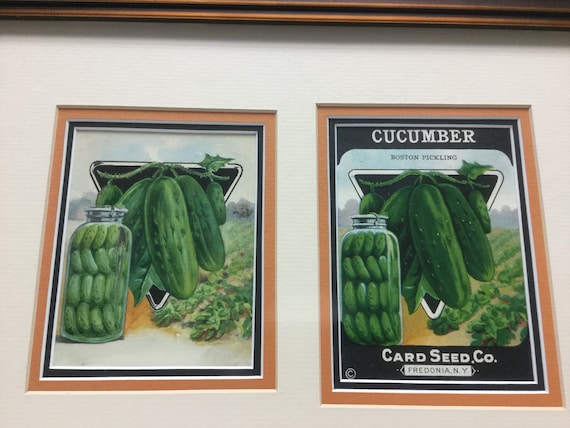This color photograph depicts a framed piece of art, elegantly presented with a brown wooden frame and off-white matting. The frame encloses two side-by-side prints, both showcasing the same detailed image with minor differences. Each print is bordered with a distinct black and orange frame. The left print features a cluster of cucumbers hanging from a green vine, complemented by a jar of pickled cucumbers in a clear glass jar situated in the bottom left. The background of this print features a pastoral scene with a sky and green fields. The right print presents a similar composition, but the cucumbers are a darker shade of green, and this version includes textual details. The top reads "CUCUMBER, BOSTON PICKLING" and underneath it, "CARD SEED COMPANY, FREDONIA, NEW YORK,” resembling a vintage seed packet. The artwork, possibly an heirloom seed advertisement, has been tastefully enlarged and framed, making it a charming addition to a kitchen or dining room.